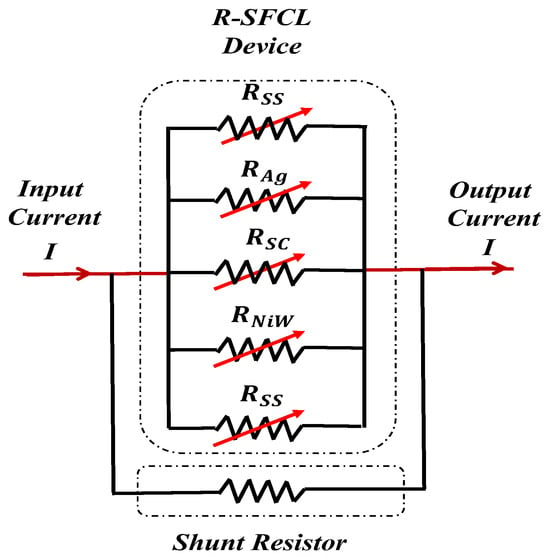This image features a detailed electrical diagram of an R-SFCL device on a plain white background, presented in black, white, and red colors. At the top, large black text labels the diagram with "R-SFCL" and "device" beneath it. Below this title, a rectangular frame is divided horizontally into five sections by black lines. Each section contains a zigzag pattern resembling electrical resistance. 

Labels indicate "input current I" on the left and "output current I" on the right. The five horizontal lines from top to bottom are marked with the following: RSS, RAG, RSC, RNIW, and RSS. A prominent red diagonal arrow stretches from the lower left, crossing each of these zigzag sections towards the upper right.

Another red horizontal arrow runs across the center zigzag labeled RSC, spanning from left to right. Additionally, there is a black bar connecting the left and right points, representing a shunt resistor, located at the bottom of the diagram. This diagram appears to depict current flow and electrical resistance within the R-SFCL device, using a combination of clear sectional labeling and directional arrows.